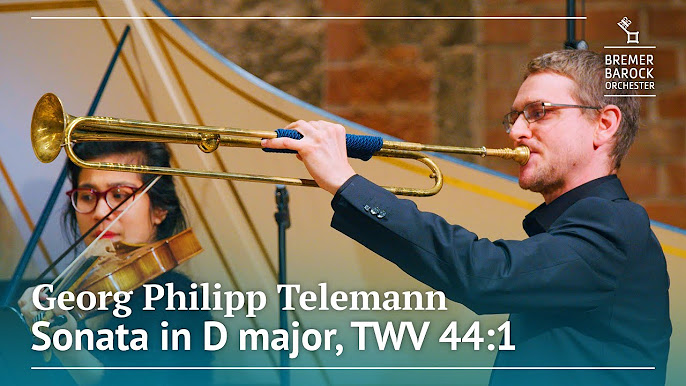In the image, a man and a woman, both wearing glasses, are positioned in front of a background featuring some brickwork. They appear to be near an open grand piano, showcasing its light oak-colored interior. The man, dressed in a black shirt and black suit with three buttons on the wrist area, holds a very long brass instrument that resembles a trumpet, possibly a baroque trumpet. This instrument also has a blue rope draped over it. The man has short hair and slight facial hair and is looking to his left. 

To his left stands a Chinese woman with deep, dark black hair styled with full, round glasses and reddish-pink lipstick. She is playing the violin and focusing intently on her sheet music. The setting appears to be a stage, possibly a promotional image for a performance. 

Above them, text reads "Bremer Baroque Orchestra," with additional details below it stating "Georg Philipp Telemann, Sonata in D Major, TWV 44:1."